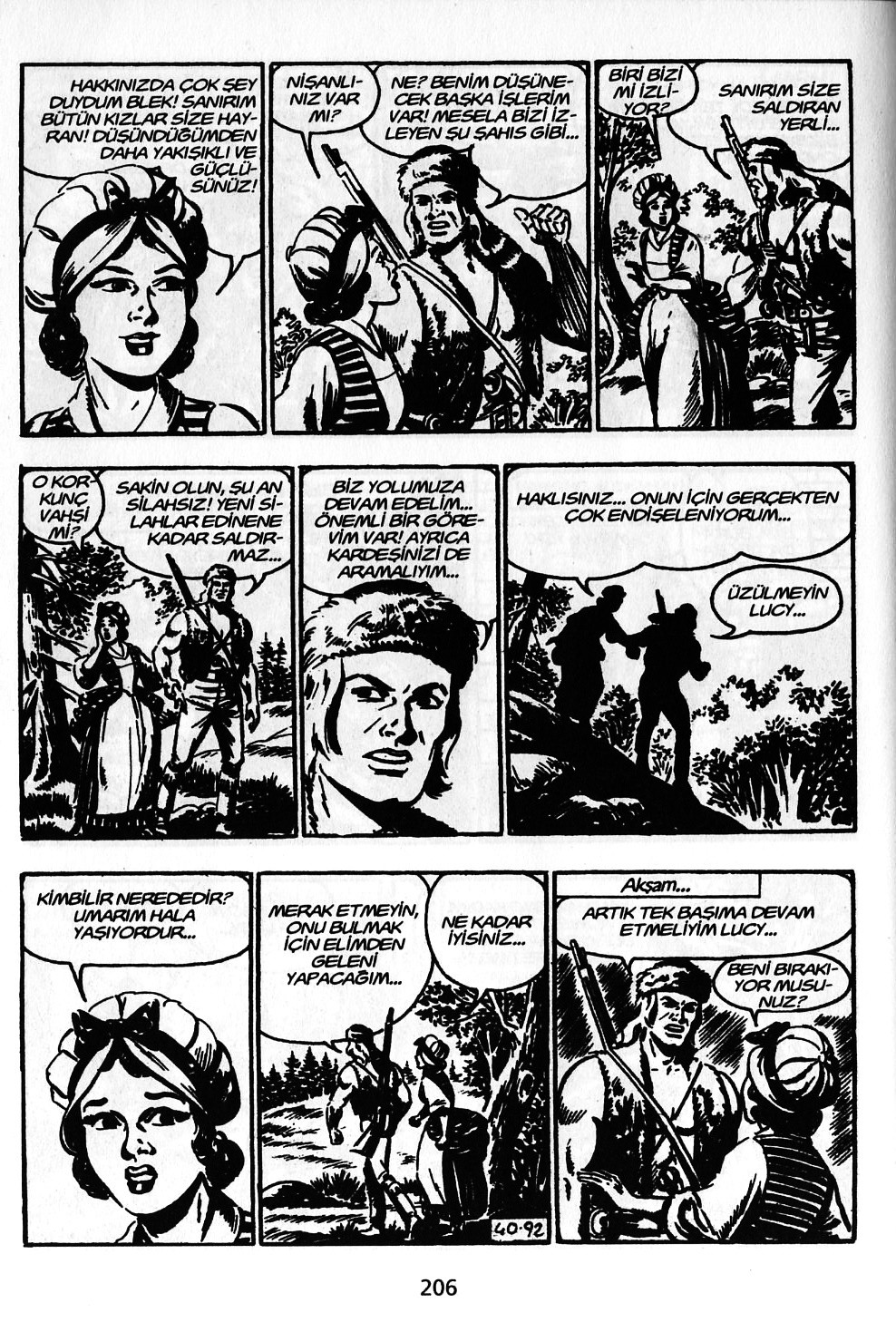This image is a black-and-white illustration, a comic book page numbered 206, featuring three horizontal panels. The page is in portrait orientation and displays vintage-style artwork. Each panel contains conversation balloons written in an unrecognized foreign language, suggesting a dialogue that is not decipherable. The scene involves a male and a female character conversing in a wilderness setting with trees in the background. The female character wears a white cap and a striped vest, while the male character, reminiscent of a historical or frontier figure, sports a coonskin cap and a feather-adorned headdress, carrying a crossbow and other weapons slung over his shoulder. The illustrations depict varying scenes of interaction between these characters throughout the panels.